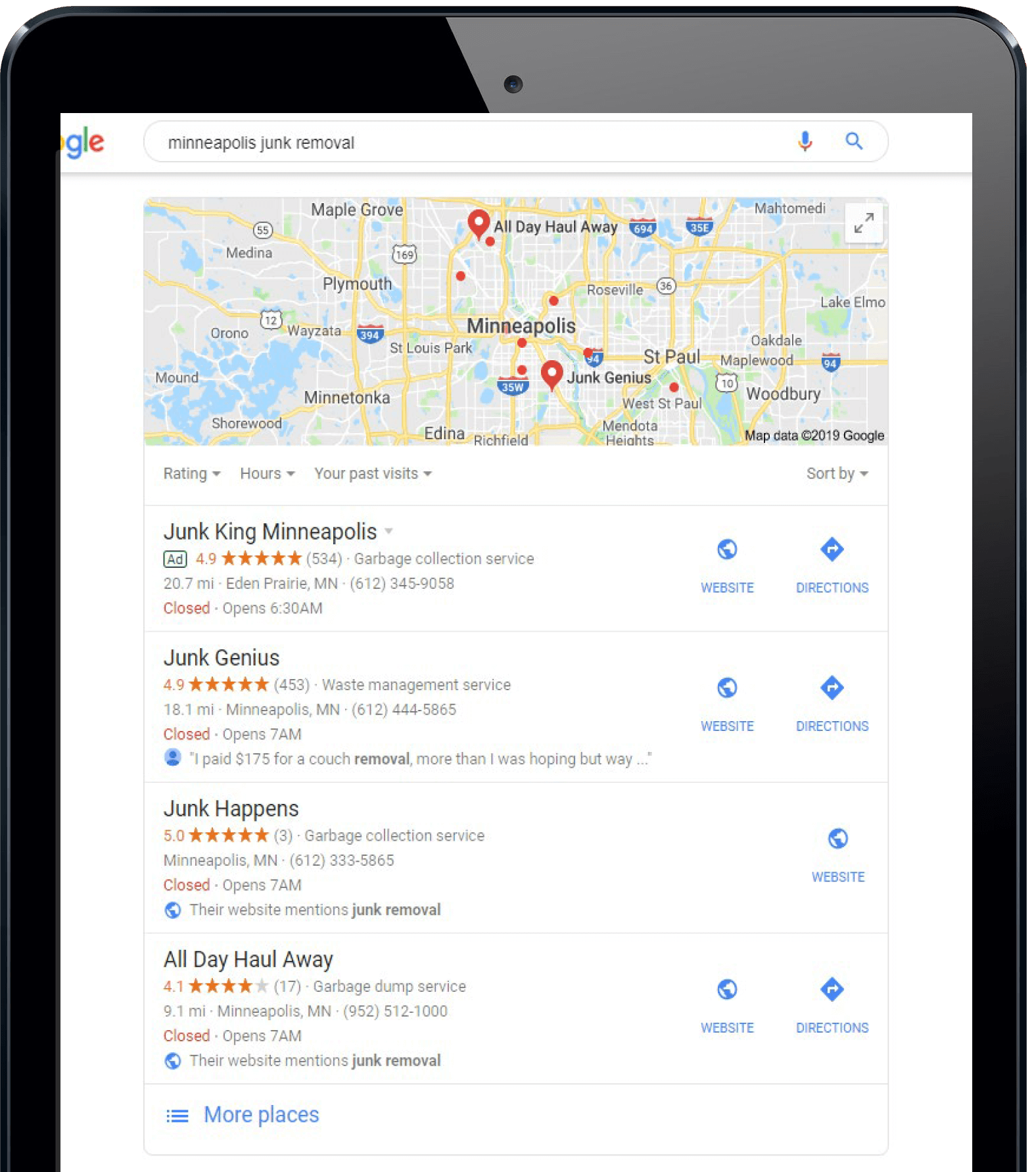The image showcases a partial screen of what appears to be an iPad displaying a Google search results page. At the top of the screen, there is a map of Minneapolis, Minnesota, with various locations highlighted. These locations correspond to search results for "Minneapolis junk removal" services. Pins on the map indicate where these services are based.

The search results list includes several junk removal services such as Junk King, Junk Genius, Junk Happens, and Holloway. Each entry in the list provides additional information, including clickable links for user reviews (highlighted in red), website access, and driving directions. Each of these services is precisely pinpointed on the map, facilitating easy navigation and choice for the user.

In summary, the image effectively illustrates a Google search for junk removal services in Minneapolis, providing a detailed view of available options and their locations on the map, complete with auxiliary information and access links.